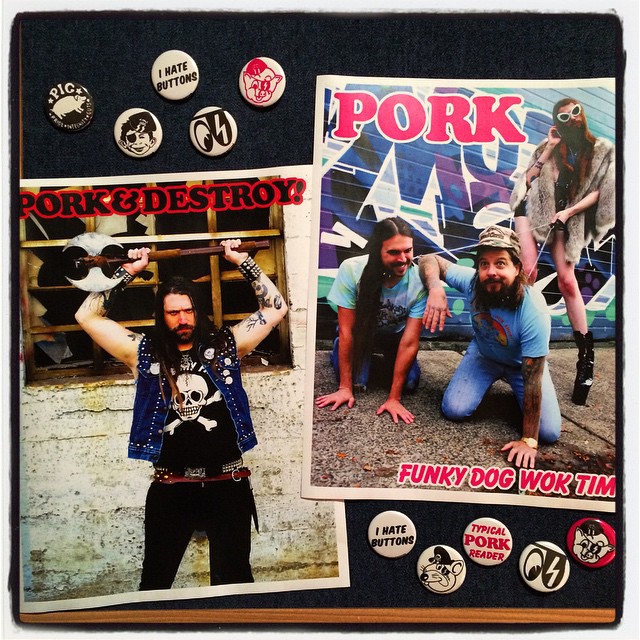The promotional flyer for the band features a striking black felt background adorned with two distinct posters of the band and an array of themed buttons. On the top left corner, the buttons include a black one with the word "pig" in white and an image of a pig, a cartoon person with an eyepatch and a peaked hat, a white button proclaiming "I Hate Buttons" in black text, a set of cartoon stylized eyeballs with the right eye sporting an eyepatch and lightning bolt, and a cartoon pig’s head in a military cap and eyepatch.

The left poster, titled "Pork and Destroy," showcases a man with tattoos on his arms, dark brown hair, and a jean jacket adorned with silver studs. He wears a black shirt with a white skull on it and holds up what seems to be a medieval hatchet, although it could be mistaken for an anvil. This man exudes a fierce demeanor, further emphasized by his long hair and black jeans, with a backdrop resembling an old medieval prison window.

On the right, the poster headlined "Pork" and captioned "Funky Dog Walk Time" at the bottom, features three men. Two are on the ground with amusing expressions suggesting laughter, while a third stands behind them wearing sunglasses. 

In the bottom right corner, additional buttons include ones with the phrases "I Hate Buttons" and "Typical Pork Reader," an image of a rat, another "Porky Pig," and an eyeball. The overall color scheme of the photos is dominated by shades of black, red, blue, and white, contrasting vividly against the black felt backdrop of the flyer.